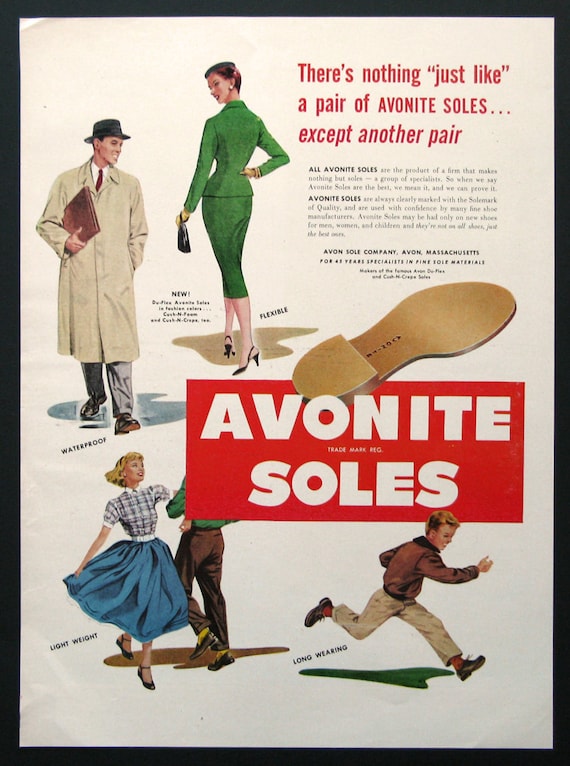This image is a detailed, full-color advertisement from the 1950s encased in a black frame. The background is off-white, enhancing the vibrant colors of the illustration. The central figure is a man in a tan trench coat and fedora, holding a satchel. Standing to his right is a woman dressed in a green dress, with text next to her that reads "flexible." Below them, a boy and girl are dancing, symbolizing "lightweight" Avanite soles. To the right, a young boy in a brown shirt and khaki pants runs towards the right side of the image, emphasizing the "wearing" comfort. The advertisement text at the upper right corner proclaims: "There's nothing just like a pair of Avanite soles except another pair." A red rectangle with white lettering prominently displays "Avanite Soles" above the running boy. Additional supportive text details the sole’s qualities: manufactured meticulously by Avon Sole Company in Avon, Massachusetts, specializing in sole materials for 45 years. The features highlighted include flexibility, waterproofing, lightweight design, and longevity, suitable for men, women, and children.